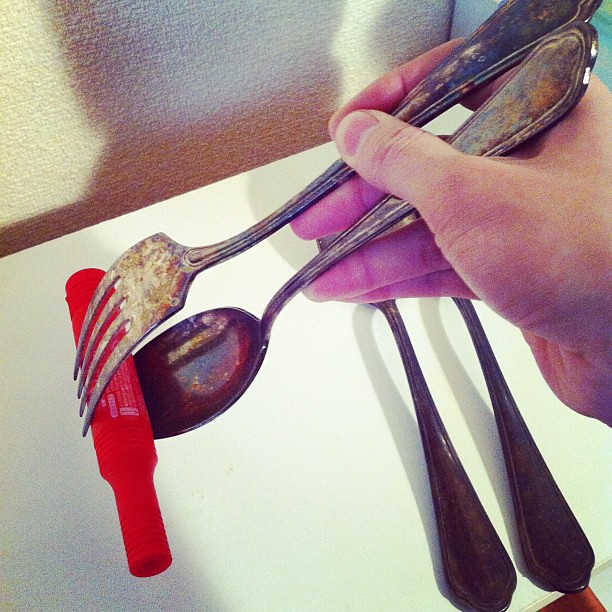In the image, a Caucasian adult's right hand is using a tarnished, rusted silver fork and spoon like chopsticks to pick up a red object resembling a magic marker. The spoon is positioned upwards and the fork downwards, meeting at their tarnished ends to clamp the marker. The fork shows more tarnish near its tines, while the spoon is more tarnished towards its bowl. The scene is set against a white table with a shadowy background, possibly a couch corner. Additionally, under the person's hand, the handles of two more tarnished silverware pieces are visible but obscured, making it unclear if they are forks or spoons. The photograph is taken from an overhead perspective, capturing the intricate details of the aged silverware and the contrasting bright red marker.